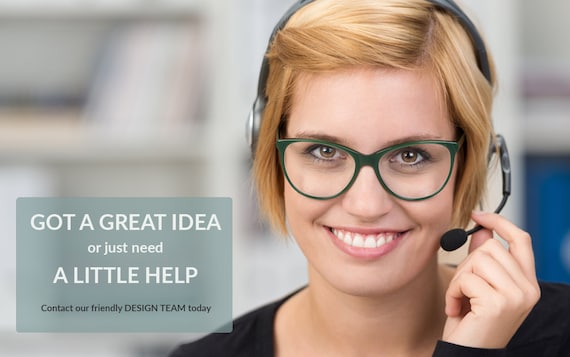In the picture, a young woman with fair skin and golden blonde hair, cut just below her ears, is smiling warmly at the camera. Positioned on the right side of the image, she sports large, gray-rimmed glasses that rest on her cheeks and has strikingly pink lips that accentuate her bright smile, revealing her teeth. Her headset, which she holds up near her mouth with her left hand, suggests she is ready to assist with a call. The woman is adorned in a black shirt, visible just below her neck and extending to her wrist. The blurred background, predominantly white, gray, and blue, provides no hints about her location or workplace. To her left, a gray rectangular sign reads, "Got a great idea or just need a little help," in white letters, with a smaller line of black print beneath it. This advertisement seems to promote a friendly design team available to help those with innovative ideas. The woman’s cheerful demeanor and professional appearance enhance the inviting and helpful message of the ad.